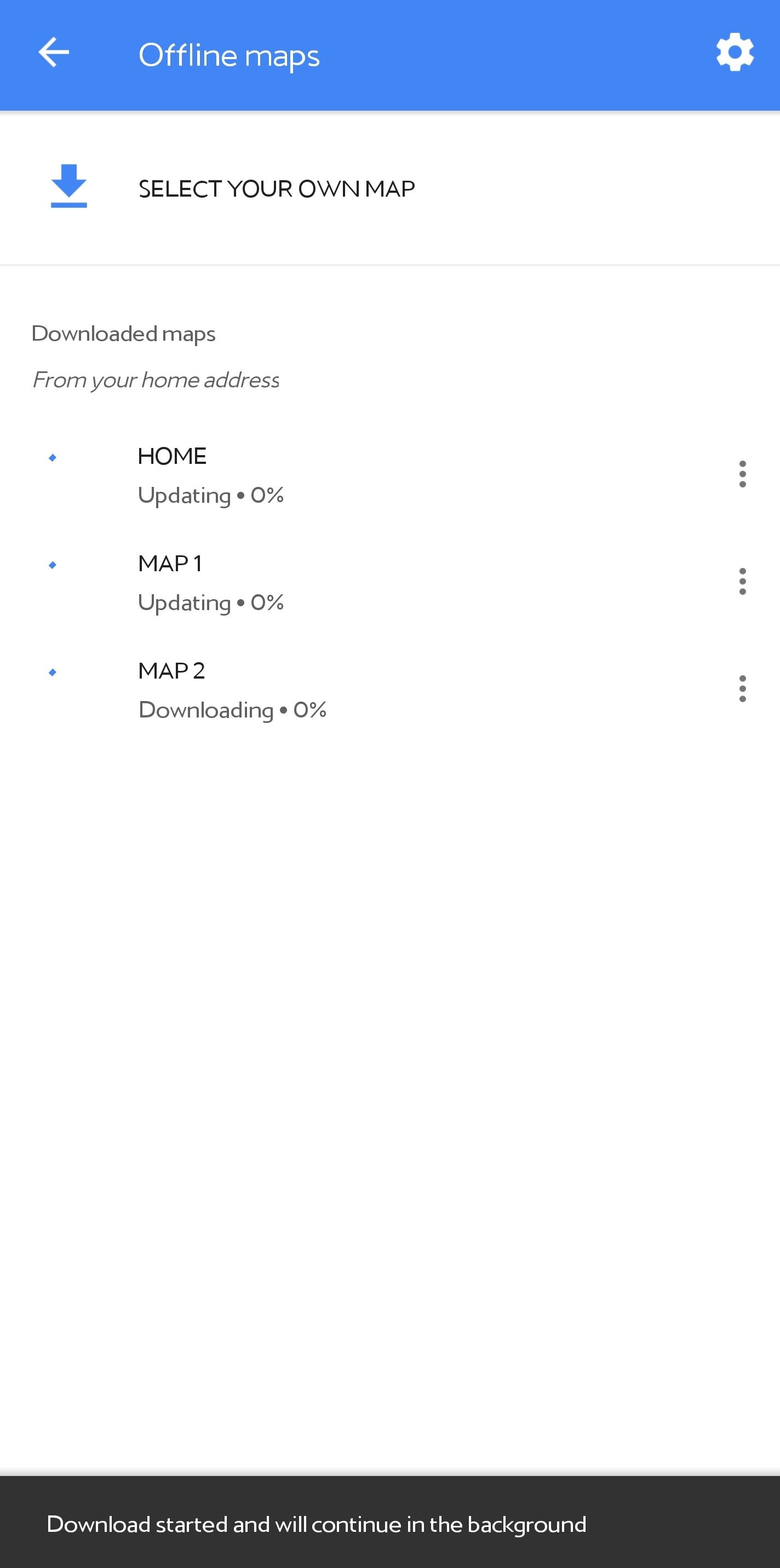The image is a screenshot taken from a computer or tablet. At the top of the screen, there is a blue banner spanning the entire width of the display, labeled "Offline Maps". On the left side of this banner, there is a left arrow icon, and on the right side, there is a white gear icon, likely for accessing settings.

Below the banner, the headline "Select your own map" is visible, accompanied by a blue downward-pointing arrow leading to a blue line also labeled "Select your own map". Further down, there is another section titled "Downloaded maps from your home address".

This section lists three maps. The first map is labeled "Home" and shows the status "Updating" with a progress of 0%. The second map is labeled "Map 1", also "Updating" at 0%. The third map, "Map 2", is marked as "Downloading", again showing 0% progress. Each of these three map entries has a small blue dot to its left. On the far right of each entry, there are sets of three vertically stacked dots, presumably for accessing additional options or settings for each individual map.

At the very bottom of the screen, a black banner with white text announces, "Download started and will continue in the background."